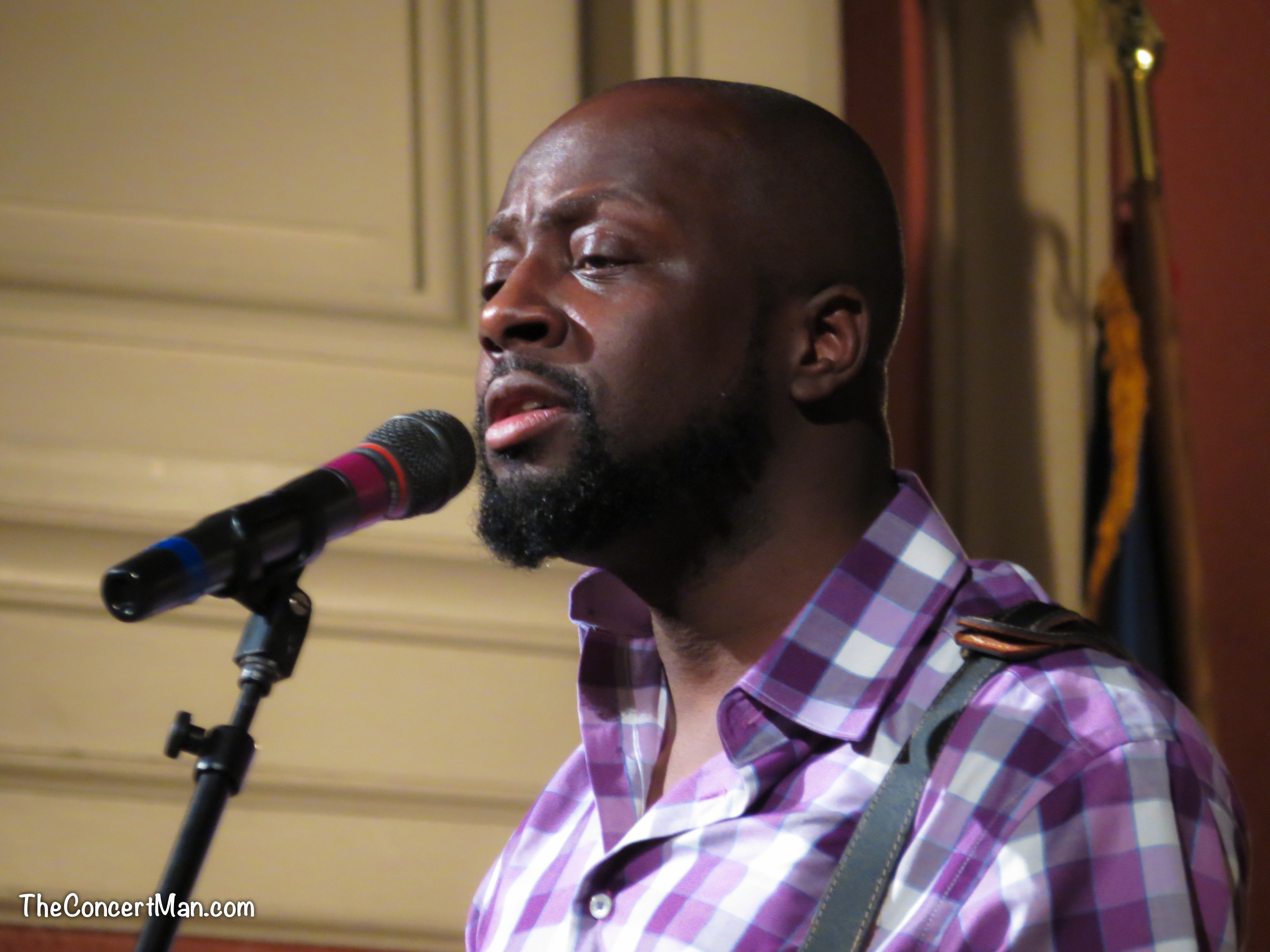In this detailed and dynamic photograph, a bald, black man is captured in the midst of singing. The image, taken from the chest up, shows him facing diagonally to the left, leaning into a distinct black microphone adorned with a red stripe at the top and a blue stripe at the bottom, positioned on the left side of the frame. The man sports a neatly groomed black mustache and beard. He is dressed in a buttoned-up plaid shirt featuring shades of purple, light blue, and white. Draped over his left shoulder is a gray strap with an orange buckle, suggesting the possibility of an instrument's support, like a guitar. The background reveals a multifaceted scene: an off-white wall with various engravings to the left, and a gold flagpole with a dark blue and orange flag hanging to the right, hinting at a formal or ceremonial setting. The combination of details in the clothing, the vibrant microphone, and the intriguing background all contribute to the richness and immersion of this close-up shot.